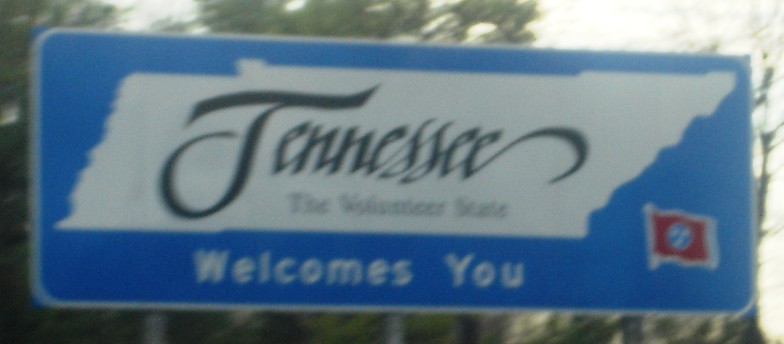This image showcases an out-of-focus road sign that welcomes travelers to Tennessee. The rectangular sign is predominantly blue, with a central white section framed by the blue background. In an ornamental black font that resembles handwriting, the word "Tennessee" stands out within the white section. Directly below this, also in black font, is the phrase "The Volunteer State." The lower portion of the sign, still in the blue section, features the words "welcomes you" written in white font. The sign conveys the message: "Tennessee, The Volunteer State welcomes you."

The blurry backdrop of the image consists of indistinct trees under a white sky, emphasizing the sign as the main focus. Additionally, there appears to be a flag, likely the Tennessee flag, integrated into the design. Despite the overall blurriness, the text on the sign remains legible, making it clear that Tennessee extends a warm greeting to all who pass by.